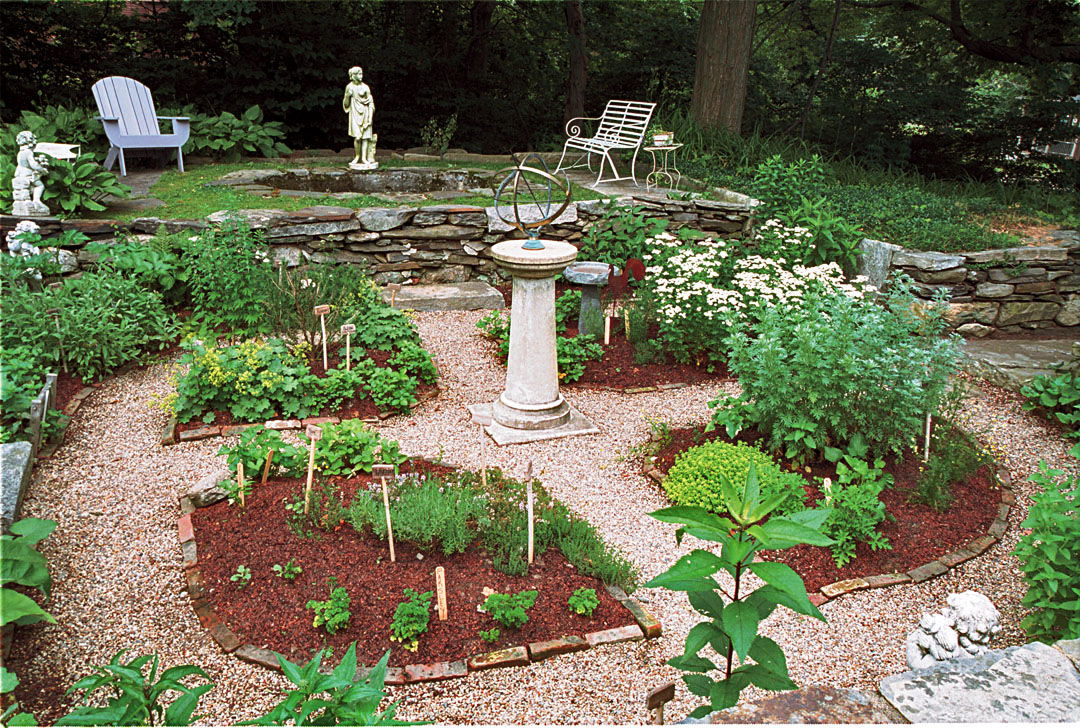This photograph captures a meticulously designed two-tiered garden with distinct elements that merge harmoniously. At the heart of the garden, a striking metal globe-like sculpture, composed of interlinked copper circles, rests atop a white Roman column in the center of a cross-shaped stone path. This path divides the garden into four verdant plots filled with plants and vegetables, each demarcated by stakes with labels. The rich red soil of the plots contrasts vividly with the white stones of the pathway. Surrounding this central feature, a low brick wall encloses the garden.

The garden's upper level features a rock retaining wall and includes additional highlights such as a couple of chairs and a side table, arranged around what appears to be either a small pond or fire pit. Another statue graces this elevated section, adding to its charm. Light-colored tan gravel covers the lower level, providing a clean and neat base. In the distance, a mature tree provides a lush backdrop, while another garden section and water feature with a circular outline add to the complex beauty of the scene. The entire layout is carefully orchestrated to create a serene, balanced, and visually appealing space.